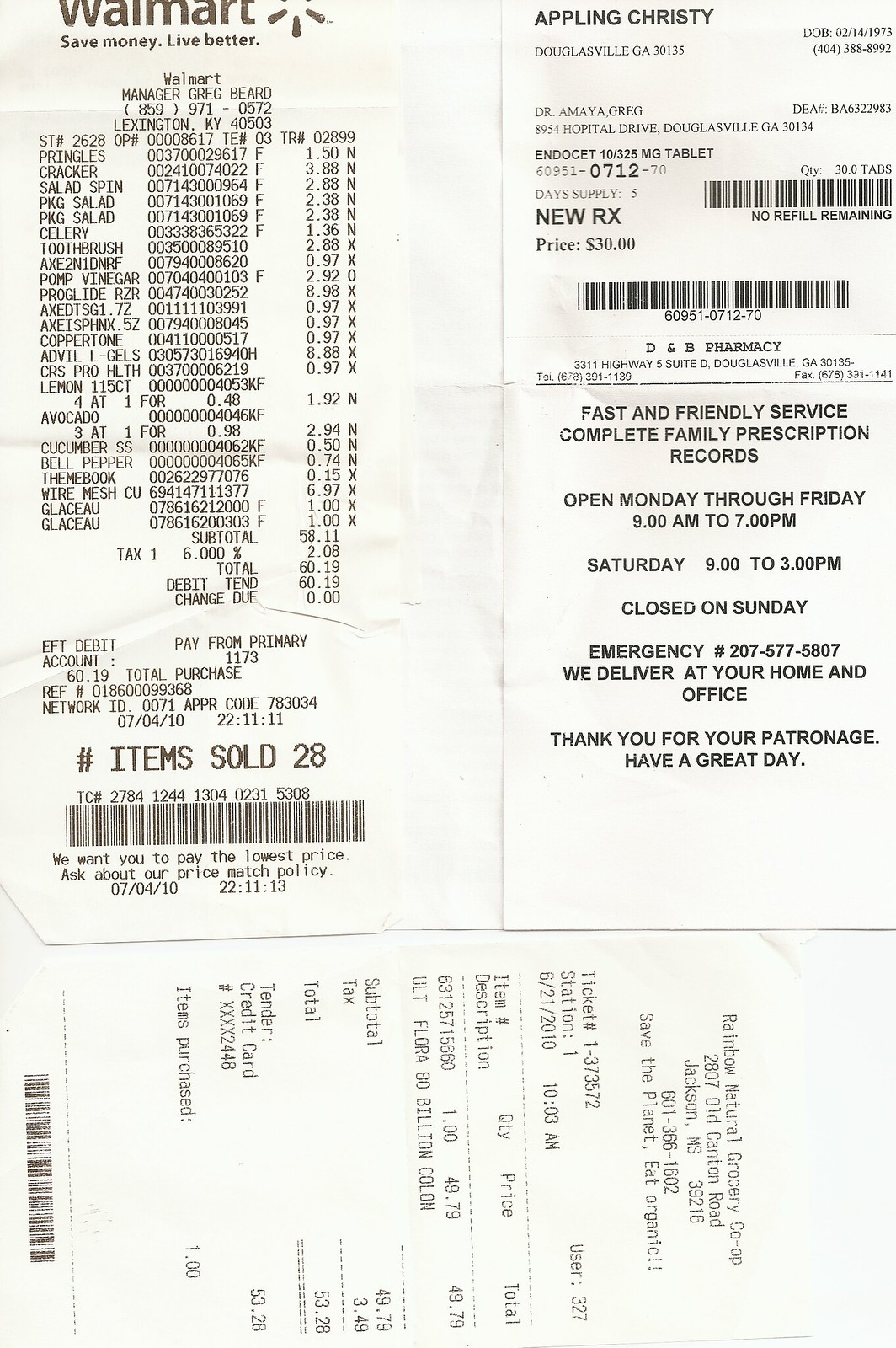This photograph vividly captures three distinct receipts against a plain backdrop, each receipt oriented in a somewhat orderly fashion. The top-left receipt is from Walmart, prominently featuring the Walmart logo at its top. Detailed lists of various purchased items follow, culminating in a noticeable statement at the bottom declaring "Items Sold: 28" in bold black text, with a barcode nestled below.

To the right of the Walmart receipt lies one from a pharmacy. This receipt, divided into two distinct sections, lists medicinal purchases including “10 325mg tablets,” highlighted by the accompanying price of $30. Beneath this transactional summary, the pharmacy advertises its fast and friendly service, complete family prescription records, and contact details, including an emergency number (207-577-5807), and operational hours which are Monday-Friday 9am-7pm, Saturday 9am-3pm.

The bottom receipt, oriented sideways with its top pointing toward the right edge of the image, pertains to the Rainbow Natural Grocery. This slightly worn and lighter receipt lists various grocery items, and finishes with another barcode at the very bottom.

Together, these receipts paint a detailed picture of a comprehensive shopping day, encapsulating visits to a major retail store, a pharmacy, and a natural grocery co-op.